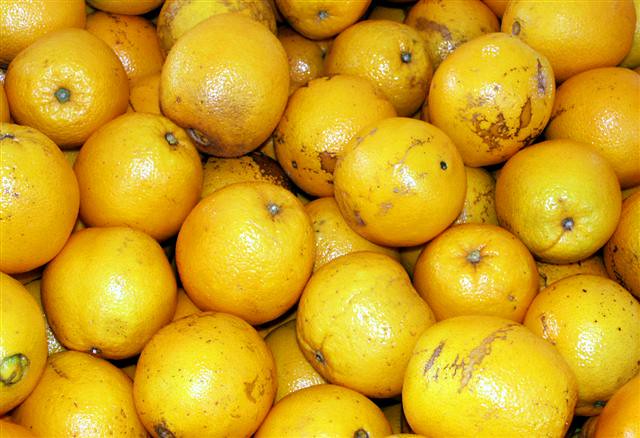This close-up photograph captures an extensive pile of juice oranges, their lighter orange hue distinguishing them from their brighter, edible counterparts. The image is illuminated with flash, showcasing a plethora of oranges piled on top of each other, filling the entire frame with at least three visible layers. The oranges are largely free of stems and leaves, indicating they've already been cleaned and processed. Among the varied sizes of the fruit, many display brown scars and imperfections, characteristic of juice oranges. Notable details include an orange with dark spots at the bottom left, another with a grayish line encircling its circumference, and an orange with a green stub protruding outwards from the left. Despite some ambiguity in exact identification, the overall appearance and coloration, with their yellowish to orange tints and white highlights, reinforce the identification of these fruits as navel juice oranges, marked by typical surface discolorations.